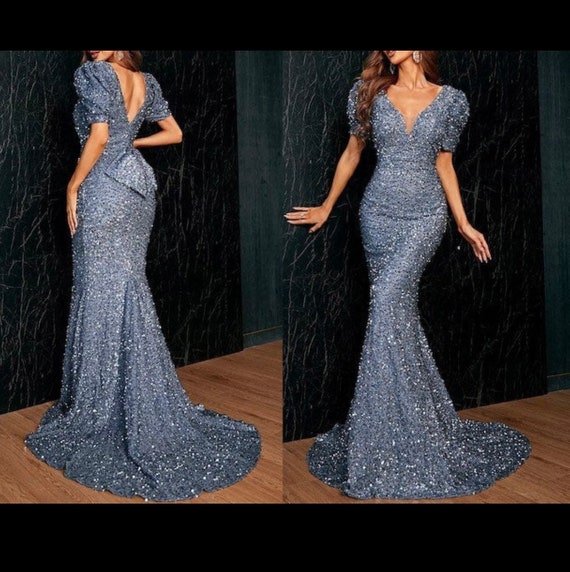The image features two side-by-side panels of a woman modeling an elegant, long, form-fitting gown. The dress, which appears to be a shimmery, dark bluish-gray or silver hue, exudes a glamorous and glittery style suitable for an extravagant event. It has short sleeves with a plunging neckline at the front and a similarly deep plunging back, both of which accentuate the model's figure. The gown flows down to the floor and fans out in a circle around her feet, giving a puddle-like effect on the hardwood floor beneath her.

In the image on the left, the model showcases the back of the dress, highlighting the detailed plunging back line. She poses with her left hand on her hip and her right hand extended to the side. To the right, the same woman displays the front view of the dress with her hands gracefully sticking out to her sides. 

The model has long brunette hair and wears large, round earrings. The background consists of a dark, textured surface, potentially resembling granite, with visible veins running through it. Wooden flooring complements the sophisticated ambiance of the scene. The top and bottom of the image are framed with black borders, adding a polished touch to the presentation. The detailed and contrasting elements create a striking and formal visual impression.